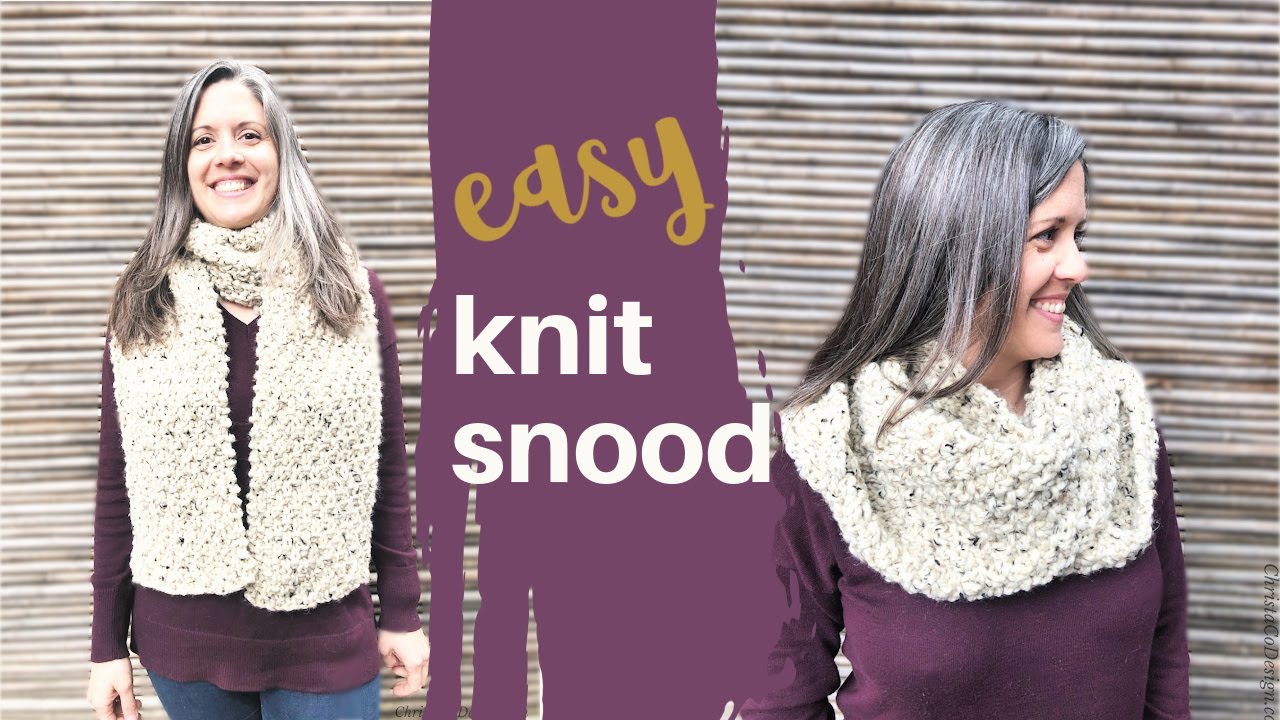The image showcases two pictures of the same woman set against a background of closely arranged wooden poles. In both photos, a vertical purple stripe with paint streaks reveals a striped pattern underneath. The stripe features the words "easy" in yellow cursive and "knit snood" in white regular font.

The woman is wearing a dark purple long-sleeved shirt and jeans in both images. She has medium-length gray hair and a warm smile, depicted with slight variations in both photos. In the left image, she stands wearing a thick white knit snood draped around her neck and hanging down to her waist, showcasing its chunky weave with some dark speckles in the fibers. In the right image, a closer shot, she has the snood styled differently, tucked around her shoulders, demonstrating another way to wear it.